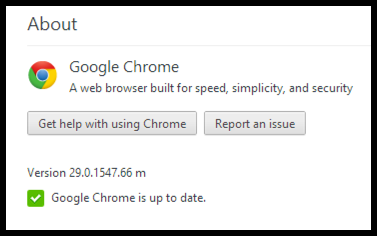This image is a meticulously cropped screenshot from the "About" tab within the settings section of Google Chrome. The top-left corner prominently displays the bold black text "About." Centered beneath this heading, "Google Chrome" is written in large, distinct gray letters. Just below, a succinct tagline in small gray letters describes Chrome as "a web browser built for speed, simplicity, and security."

Further down, to the left, a long, gray rectangular bar features the text "Get help with using Chrome" in small black letters. Adjacent to this bar on the right is a square box labeled "Report an issue." At the bottom left corner of the screenshot, the version number of the browser is displayed. Beside this, a green box with a checkmark contains the confirmation message that "Google Chrome is up to date," also in small black letters. 

The entire screenshot is outlined by a thin black border, signifying its cropped nature from the original settings page.